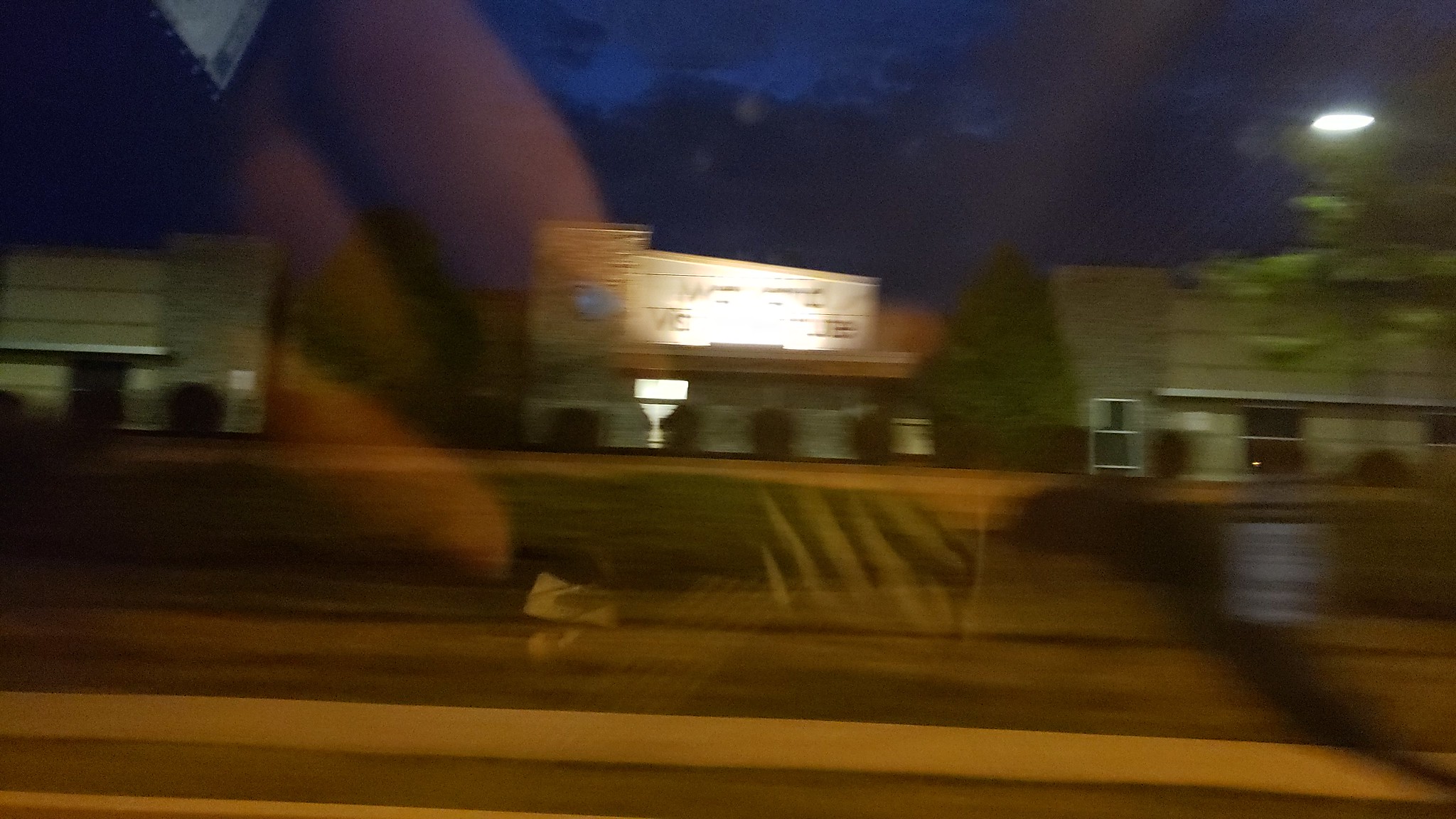This image, positioned wider than it is tall, captures a dimly lit residential area at twilight, likely through a window from a moving vehicle, possibly a bus. Blurriness and significant glare dominate the photograph, with semi-transparent reflections of fingers and a computer screen adding to the chaotic composition. In the lower section, a road with a visible white line and curb is present. A chain-link fence extends in front of three one to two-story houses with paneled fronts, some brick siding, and bushes in the yard. The first and third houses are dark, while the second, illuminated house features an unreadable lighted sign on its roof and multiple doors. Flanking the lit house are trees, and a square white sign hangs on the fence to the right. The sky above is a dark purple, suggesting the last vestiges of light, and a lone street light shines on the scene from the far right.